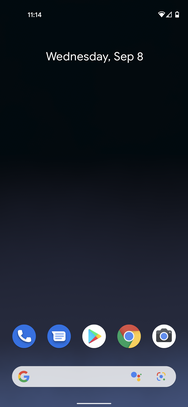This image is a portrait-mode screenshot of a cell phone home screen with a minimalist design. In the upper left corner, the time reads "11:14," while the battery icon in the upper right corner is approximately halfway filled. Just below, the date is displayed as "Wednesday, September 8th" in a straightforward white font.

The background of the screen starts as a very dark black at the top, gradually lightening to a dark, almost light black shade as it descends. Further down, the shade transitions to a navy blue by the bottom of the screen. 

Centered on the lower portion of the screen are five prominent icons arranged in a row: 
1. A blue circle with a white phone icon, representing the phone app.
2. A blue circle with a white speech bubble icon for messaging.
3. A white circle with a colorful Google Play Store icon.
4. The multi-colored red, yellow, green, and blue circle representing Google Chrome.
5. A white circle with a camera icon.

Below these icons is a Google search bar, distinctive with its small "G" logo on the left end and a rounded square icon on the right end, which features segments in red, yellow, green, and blue with a central blue dot, possibly indicating an image upload function. Next to this icon is another featuring a circle overlaying what resembles a small yellow bottle, which might represent Google's new AI feature.

Overall, this clean and modern home screen design balances functionality with an aesthetically pleasing gradient background.